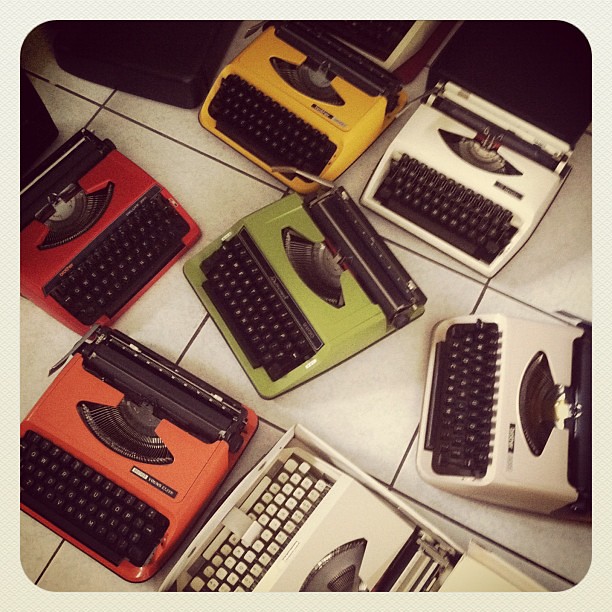This is a top-down photograph of seven vintage typewriters, each with a distinct colored shell, arranged on large white floor tiles. Starting from the top left, there is a black typewriter facing towards the right. To its immediate right is a yellow typewriter with black keys. Next to that, to the right, is a white typewriter with black keys. The typewriter in the center of the image is lime green with black keys and a black roller at the back. Below it, towards the left, is a red typewriter with black keys, also facing right. Adjacent to this, to the right, is an orange typewriter with black keys. At the very bottom center of the image sits another white typewriter with white keys. All the typewriters appear to be the same model, differentiated only by their colorful exteriors. This photograph is framed within a cream-colored card with a textured pattern of crossed lines, and the card itself has curved corners.